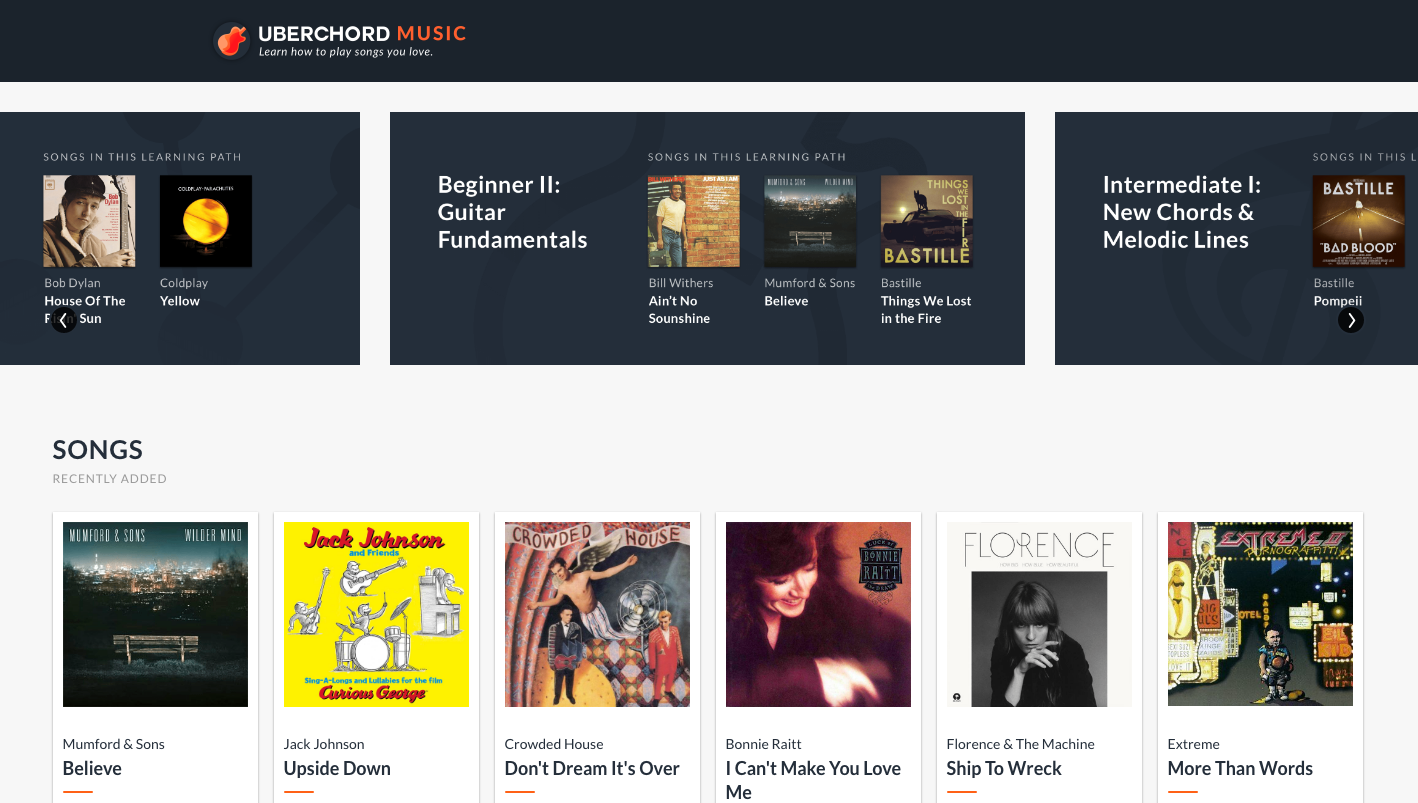This is a detailed caption for the image provided:

"The screenshot captures the interface of a music website titled 'Record Music.' At the top of the interface, the website's name is prominently displayed. Below the title, there are various categories or genres that organize the songs available on the platform. Toward the bottom section, a list of song titles is visible, including 'Believe,' 'Upside Down,' 'Don't Dream It's Over,' 'I Can't Make You Love Me,' 'Ship to Wreck,' and 'More Than Words.' The layout suggests a user-friendly browsing experience, with a clear organization of musical content for easy navigation."